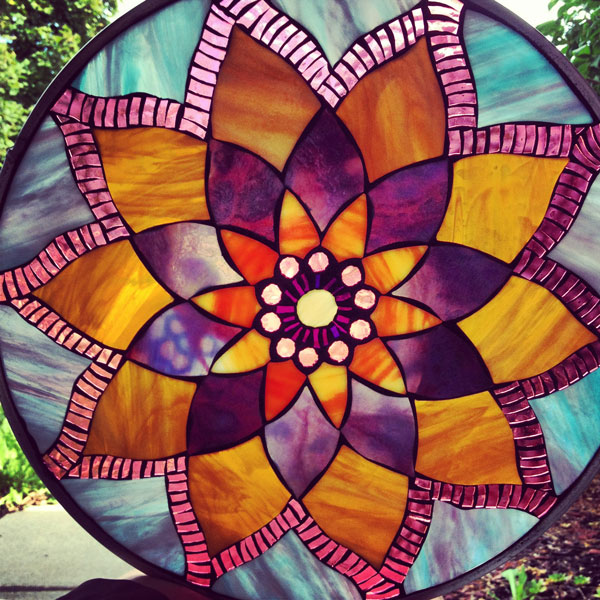This is a photograph of a towering garden decoration, at least seven feet tall, featuring an intricate stained glass design. The centerpiece is a large, circular metal frame holding a stunning flower pattern. The flower, composed of multiple layers of petals, ranges in colors including gold, orange, purple, fuchsia, and white, with black lines delicately separating many petal edges. The innermost circle of the flower includes a mix of yellow and orangish-red hues, expanding outwards to purple and fuchsia petals. The outermost layer features smaller rectangles of fuchsia pink, again separated by black lines, extending to the edges of the blue, purple, and white streaked background. Beneath this vibrant artwork, the ground shows a mix of dirt and grass, indicating its outdoor setting. In the background, it's a sunny day with green trees and foliage visible, adding a natural contrast to the colorful stained glass display.